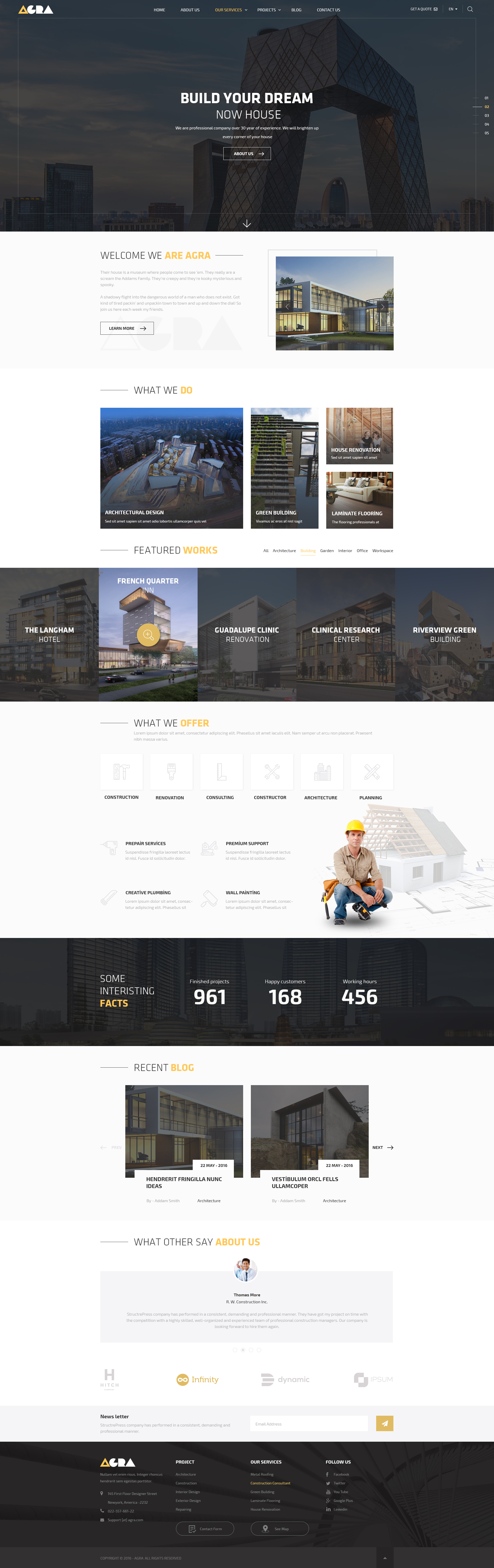The image depicts a lengthy web page composed of various sections. At the top, there is a banner featuring a backdrop of multiple structures with a sky towards the left, dotted with wispy white clouds. The bold, uppercase text "BUILD YOUR DREAM" is prominently displayed in white across the middle of the banner. Beneath this, there is thin white text that is difficult to read, followed by even smaller white lettering.

Transitioning into a white section, the heading reads "WELCOME WE" in capitalized dark gray or black font, flanked by the words "ARE A G R A" in orange towards the right, though the exact text is unclear. Adjacent to this text, an area shows several buildings under a blue sky with some clouds to the right. This section features two editable fields or paragraphs beneath the top text.

Scrolling down, there's a button with a white background, a black border, black text on the left, and a black arrow on the right. Following this, a heading states "WHAT WE DO," with "WHAT WE" in black and "DO" in orange, separated by a line. Below this heading, there are four distinct images: the first, a long rectangular picture possibly depicting sand with a blue area at the top, and two smaller, indistinct images to the right.

The page continues with a lengthy menu overlaying images in the background, featuring centered white capitalized text and smaller white lettering below. Finally, in the bottom-right corner of another white section, a construction worker is visible, kneeling while wearing a yellow hard hat, a long-sleeved beige shirt with rolled-up sleeves, and blue jeans.